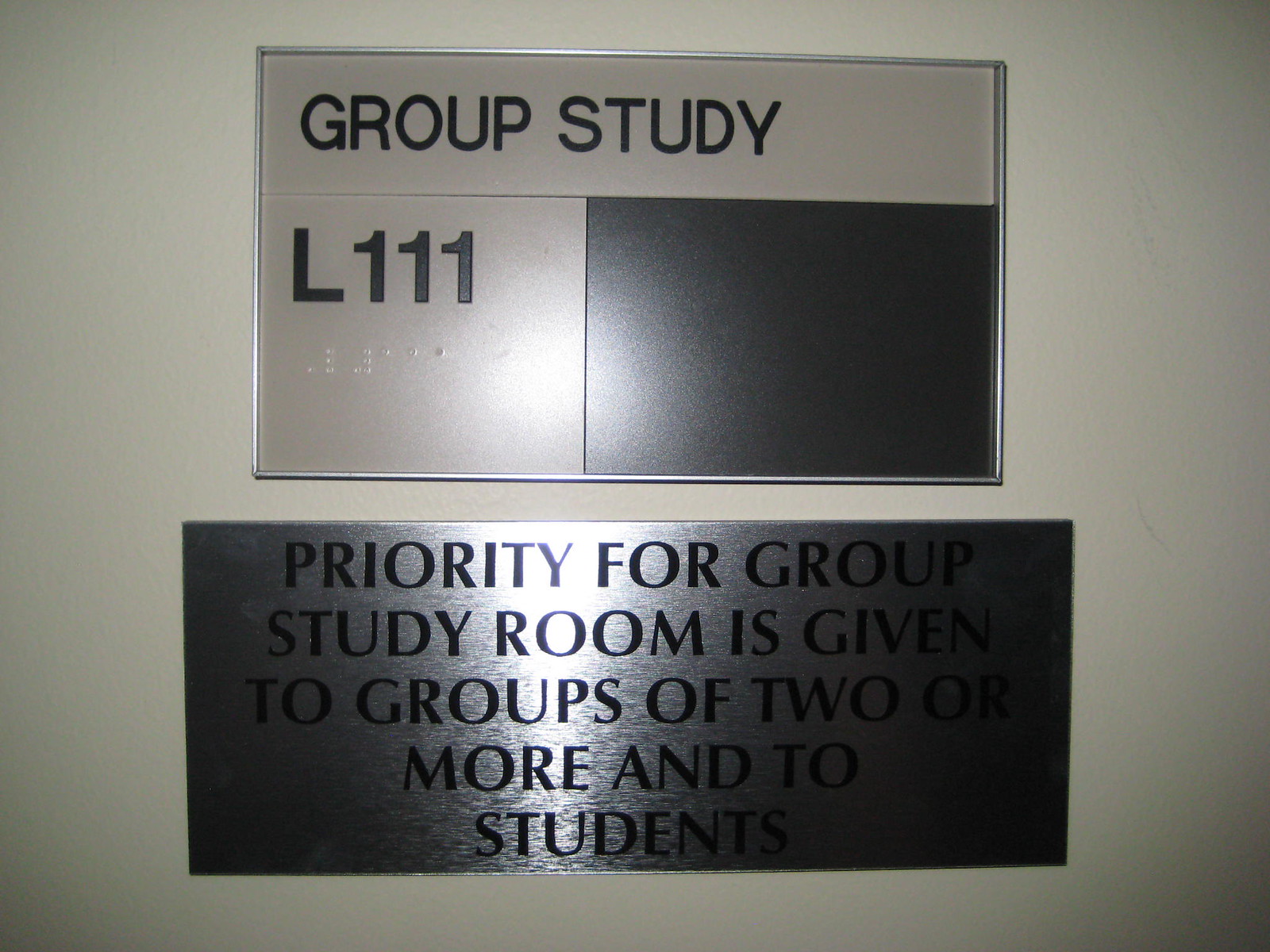This image depicts two informational signs displayed on a solid white wall, typically found in an educational institution such as a university or college. The top sign features white with black letters and reads "Group Study," followed by the room number "L111," and includes braille text for accessibility. Positioned directly below, the second sign is crafted from brushed metal with black letters, stating "Priority for group study room is given to groups of two or more and to students." These signs likely indicate the regulations and identification for a group study room, meant to ensure that the space is used appropriately by small student groups rather than individuals.